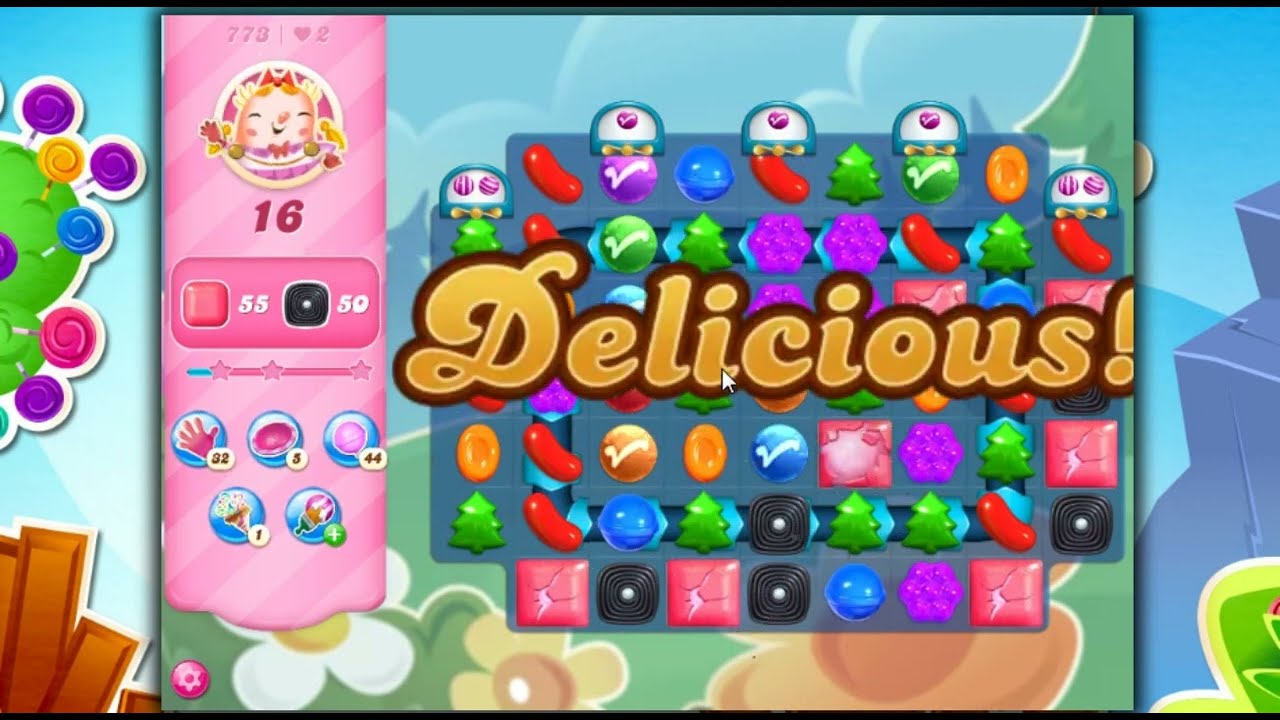The image is a vibrant screenshot of a mobile video game featuring a colorful, sky-themed background with clouds, flowers, staircases, and various multicolored objects such as fruits, beans, and chocolates. Prominently displayed in the center, the word "Delicious" is creatively rendered in large orange bubble letters with an exclamation mark. 

On the left side of the screen, a pink vertical bar acts as a scorecard, showing a score of 773 at the top, accompanied by a heart icon and the number 2. Below this, there is a profile picture of a cute animated character with a red bow on her head, and the number 16 positioned just beneath the character.

Further down, there's a box with a pink square and a black square containing the numbers 55 and 50, respectively, alongside a camera icon. Below this is a horizontal progress bar that has three stars at interval points, starting to light up in blue from the left just before reaching the first star.

At the bottom, five circular icons are arranged in a pattern. The icons include a hand with the number 32, a blue or purple button with the number 5, a lollipop with the number 44, an uncertain icon with an upside-down triangle of curlicues and the number 1, and a green plus circle with purple and white stripes. The bottom corner also features a settings button.